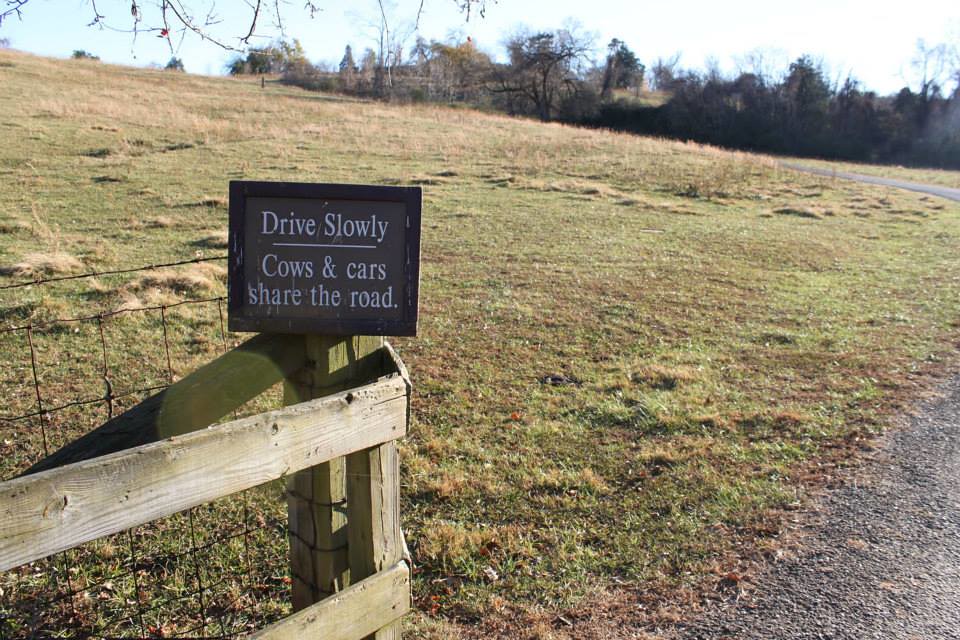The image depicts a serene country setting with a large field of mixed green and tan grass dominating the landscape. A wooden and wire fence, featuring a prominently open gate, stretches across the foreground. A rusty rectangular sign attached to the gate reads, "Drive slowly—cows and cars share the road," underlined in white for emphasis. To the right, a dirt roadway, dark brown and winding slightly to the left, disappears into the distance. The background features a bright blue and white skyline, dotted with trees, and the faint outline of a building is visible on the top left. Overhanging branches add a touch of natural framing to the rustic, tranquil scene.